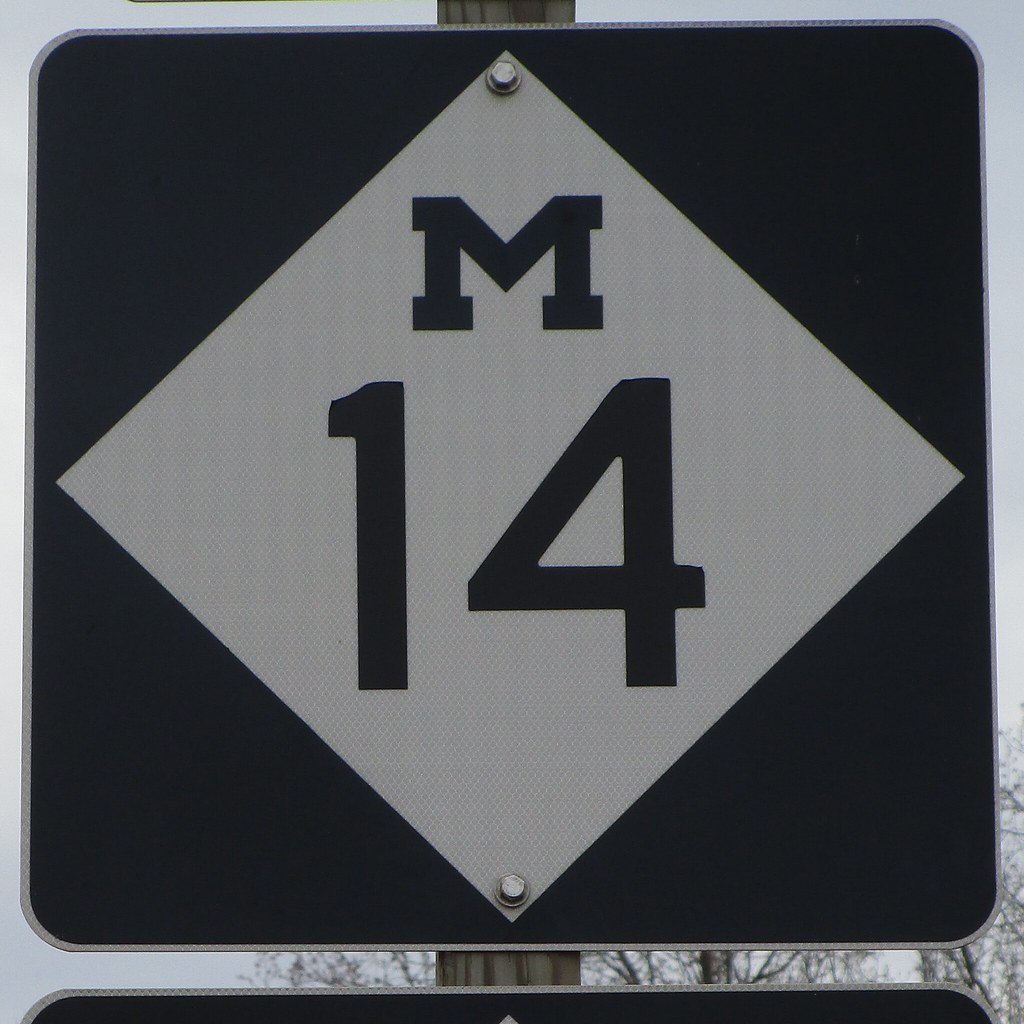The image features a close-up of a road sign mounted on a wooden pole. The primary sign is a black square with rounded corners, subtly outlined in silver. Dominating the center of the square is a white diamond, containing a boldly printed black uppercase "M" and the number "14." The scene is set against a backdrop of overcast skies, tinging the atmosphere with a melancholic gray hue. Partially visible beneath the main sign is another sign, although only its top part is in view, making its full content indiscernible. Branches and trees partially frame the background, enhancing the somber and muted ambiance of the day.